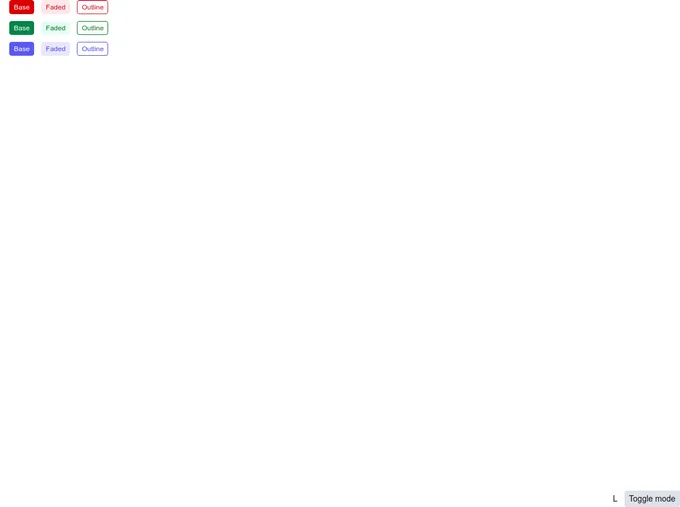The image showcases a website with a predominantly white background, maintaining a clean and minimalistic aesthetic. 

At the top, there is a three-by-three grid with distinct colored squares. 

- The first row features a solid red square with softened edges and rounded corners, containing the word "Base" in white text.
- Adjacent to it is a faded pink square, subtler in hue, with the inscription "Faded" in red, featuring a capital "F".
- Completing the first row is a white square outlined in red with the word "Outline" in red capitalized text "O".

The following rows replicate this pattern with different colors:
- The second row displays the same arrangement, but in green: a solid green square labeled "Base," a faded green square labeled "Faded," and an outlined green square labeled "Outline."
- The third row uses purple to mirror the pattern: a solid purple square labeled "Base," a faded purple square labeled "Faded," and a purple outlined square labeled "Outline."

On the right side of the grid, approximately halfway down the page, there is a small gray button with the text "Toggle Mode" in black print, featuring a capital "T".

This meticulous arrangement ensures that each color category is represented consistently across the rows, highlighting the different visual styles ("Base," "Faded," and "Outline") within each color group.